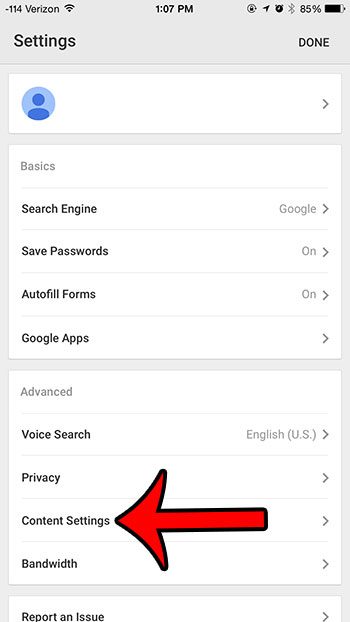This is a detailed screenshot of an Android phone's Settings app, taken at 1:00 PM with the battery level at 85%. At the very top of the screen, the Settings title is displayed in the upper left corner, accompanied by a 'Done' button in the upper right corner. The toolbar reveals the time and battery percentage.

The screenshot showcases two main sections within the Settings page: Basic and Advanced. The Basic section comprises options such as Search Engine, Save Passwords, Autofill Forms, and Google Apps, all presented as dropdown menus.

Below the Basic section lies the Advanced section, which includes Voice Search, Privacy, Content Settings, and Bandwidth. A large red arrow, hand-drawn, directs attention specifically to the Content Settings dropdown menu within the Advanced section. This arrow seems to be part of an instructional guide embedded in the screenshot, intended to emphasize the Content Settings feature for the viewer.